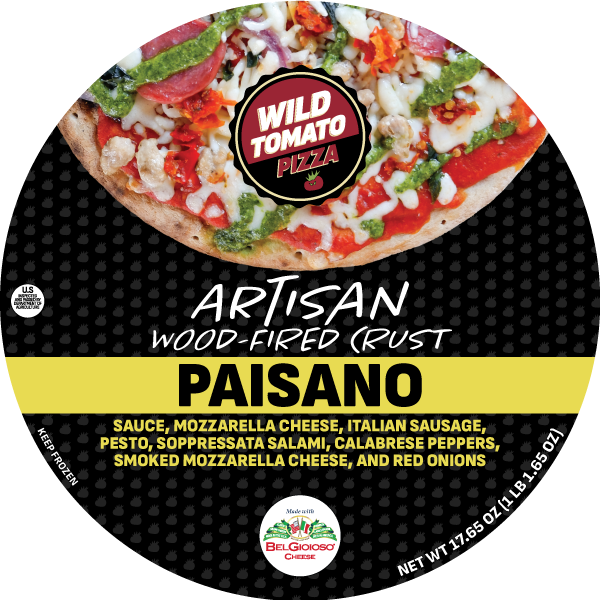The image is a detailed advertisement for a frozen pizza by Wild Tomato Pizza. The circular label highlights the artisan wood-fired crust Paisano pizza. The top portion showcases a tempting visual of the pizza, which appears to be topped with sauce, mozzarella cheese, Italian sausage, pesto, soppressata salami, calabrese peppers, smoked mozzarella cheese, and red onions. A prominent feature includes the text "artisan wood-fired crust" with a notable yellow horizontal stripe reading "Paisano." The logo of Wild Tomato Pizza, half red and half black with a tomato underneath, is also displayed. Additionally, there are smaller, unreadable logos, a label indicating "keep frozen," and a weight specification of 17.65 ounces (1 pound, 1.65 ounces). The detailed imagery and comprehensive list of ingredients create a mouth-watering presentation of this gourmet frozen pizza.